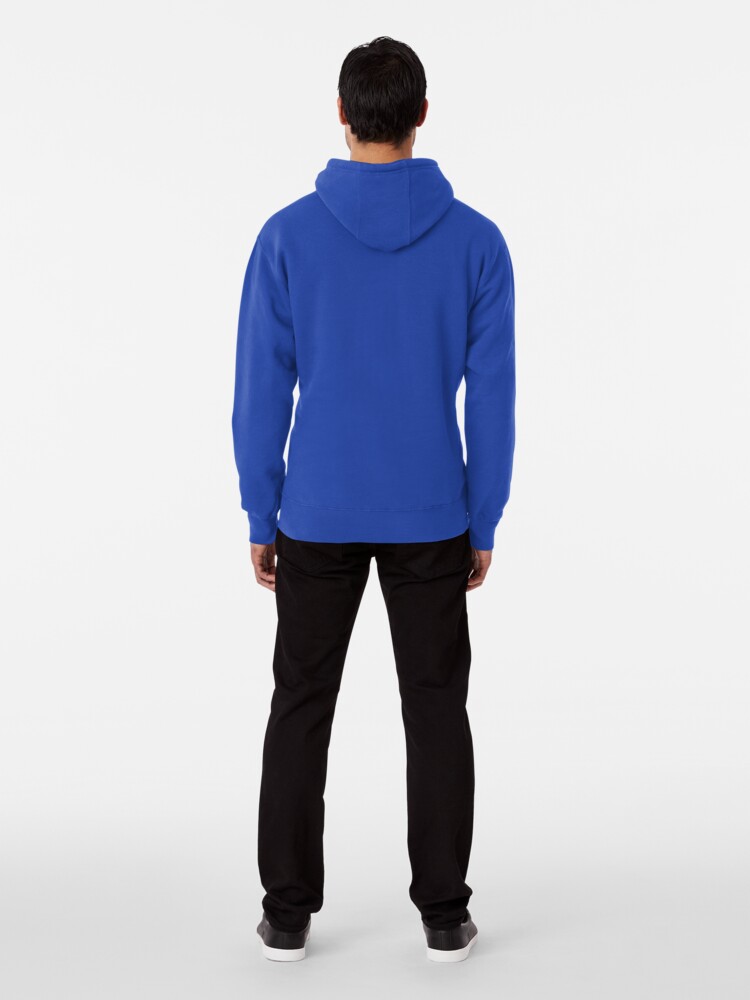This image depicts a man standing with his back to the camera against a background that transitions from white at the top to a lighter gray at the bottom. The man has short, sharp black hair and is dressed in a blue hoodie with a seam down the middle of the hood. The hoodie is paired with black pants that reach down to his ankles, where there’s a slight excess of fabric. He is also wearing black leather sneakers with white rubber soles, which appear a bit shiny. The man's stance is casual with his legs slightly spread apart and his arms hanging straight down by his sides. There are no other elements or people in the image, suggesting it may be a stock photo meant to highlight the apparel.